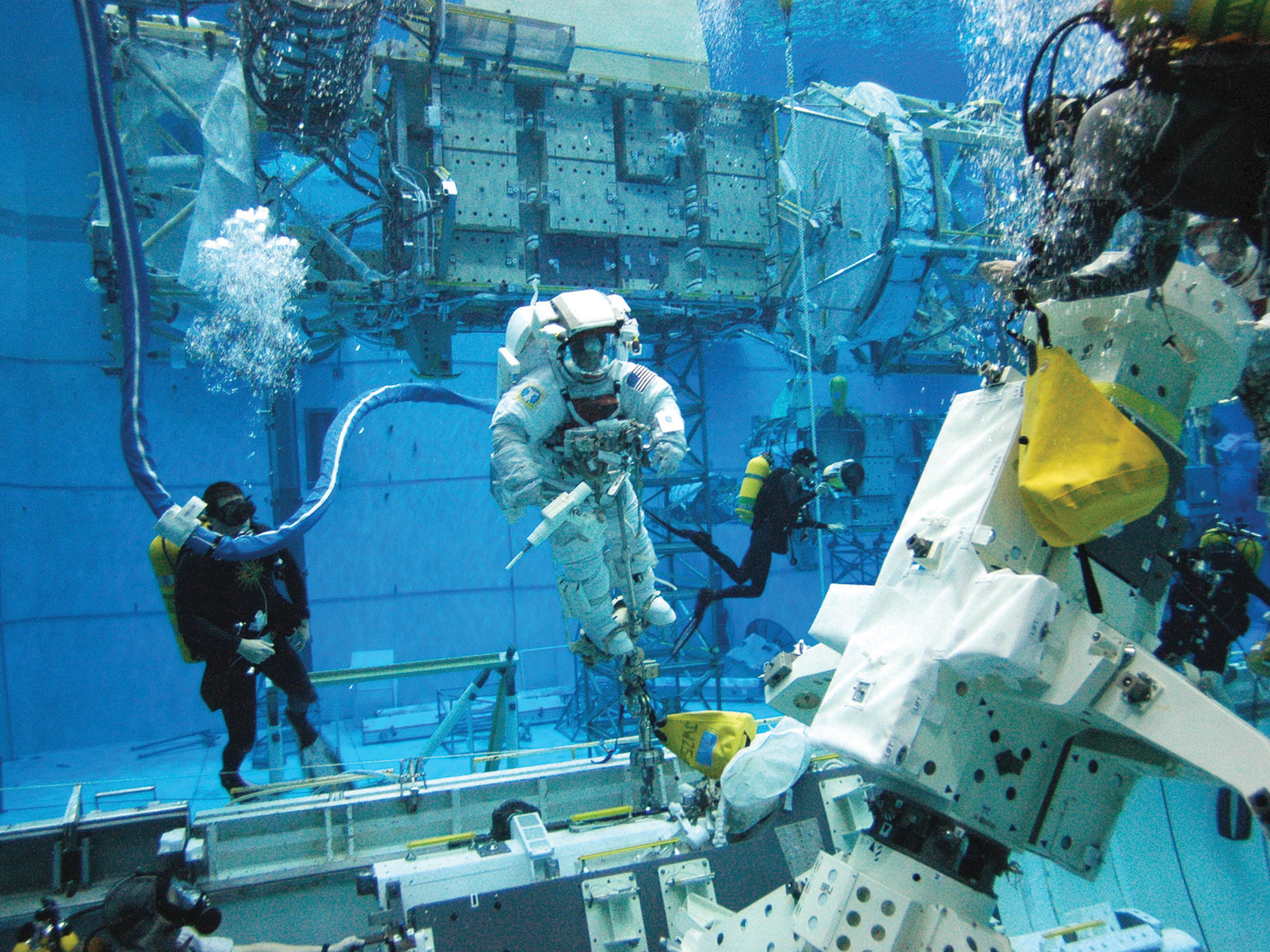In an underwater training facility run by NASA, a white-suited astronaut equipped with a helmet and a backpack is engaged in a simulation exercise. The astronaut, holding a tool, is working on equipment that resembles structures found on the International Space Station or possibly an old space shuttle bay, characterized by multiple nuts and bolts. His feet are secured in stirrups weighed down by a yellow bag, likely attached to the bottom of the tank. Surrounding him are five scuba divers, clad in black wetsuits with yellow oxygen tanks, helping facilitate the training. The divers' air bubbles are visible, rising to the surface of the water, which is the predominant blue hue in the scene. This setup, featuring cylindrical and box-shaped components, emulates the conditions of weightlessness in space, enabling astronauts to practice their tasks in a simulated environment.